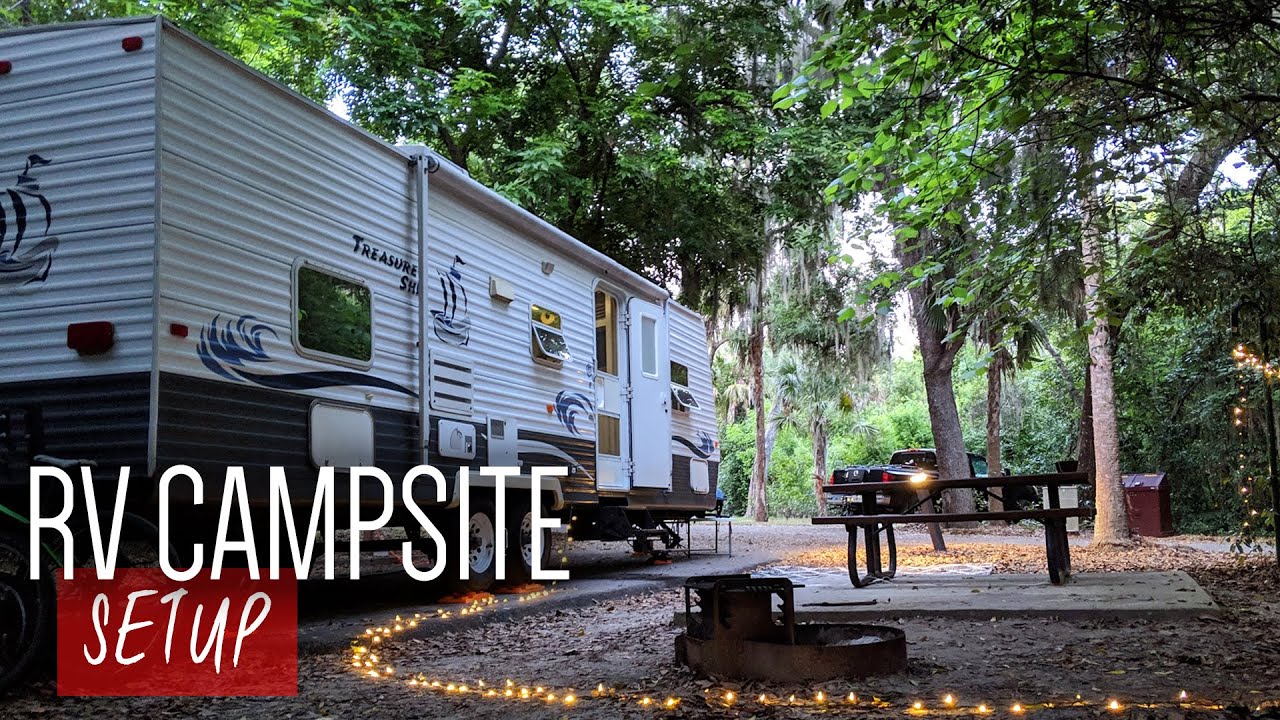The image is a detailed photograph of an RV campsite presented in a horizontal rectangle format. Dominating the left side of the image is a large camper with its front end extending towards the middle. The camper is mostly white with brown accents at the bottom and features various emblems, including black writing and a depiction of a wave and a ship. Visible elements include a window at the back, a door towards the front, and possibly another window on the side. The camper appears slightly elevated, likely resting on its wheels.

String lights are artfully draped around the campsite, forming a semi-circle around a dirt area with a central fire pit, though the fire is not lit. Adjacent to this dirt area is a concrete slab with a wooden picnic table upon it. Further into the background, trees frame the scene, with one large tree extending out of the image at the top right and another slightly smaller tree on the left. Behind these trees, a vehicle, resembling a truck, is partially visible.

In the bottom left-hand corner of the image, large white text reads "RV Campsite," and just below this in a red box, the word "SETUP" is prominently displayed in white letters.